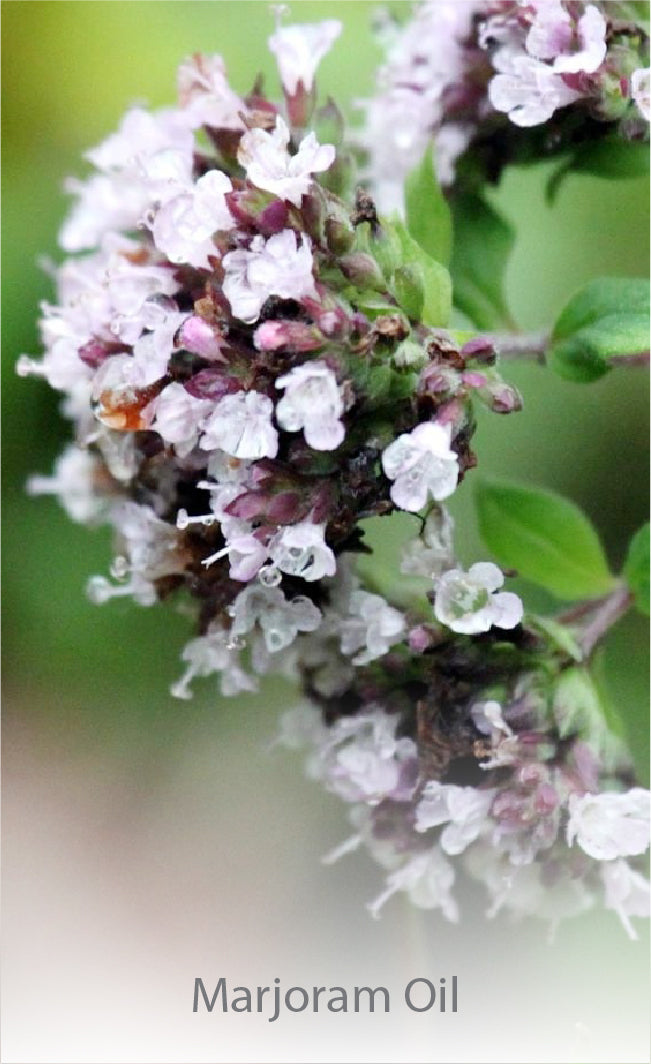In this image, nature takes center stage with a low-quality, grainy photograph of a flowering plant. The composition features a cluster of delicate blossoms, predominantly light pink, located towards the upper right of the frame, yet some flowers extend towards the center. The more mature buds interspersed among them are darker in color and appear slightly hairy. The stems of the plant reveal pointed ovate leaves further down. The flowers collectively exhibit tiny translucent petals, each facing left, and some blooms exhibit bilabiate symmetry, mirroring each other if cut in half. One flower on the left side shows signs of browning or yellowing. The blurred, gray-toned background suggests an outdoor setting, likely a garden or wilderness. At the bottom of the image, the grey text reads "Marjoram Oil."